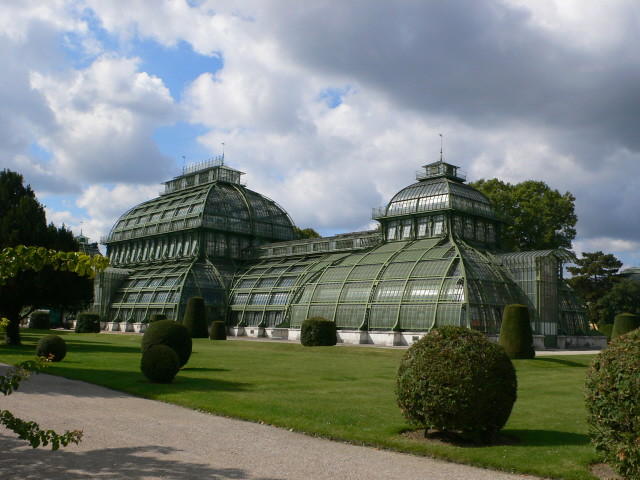The photograph showcases a unique and eye-catching building predominantly made of glass and metal, with a notable dome shape featuring rounded and thinner upper edges. The structure appears expansive, possibly housing a conservatory, with light green bars accentuating its glass panels. The building is anchored by a solid white line at its base, likely a cement foundation. Dominating the foreground is a well-manicured green field dotted with variously shaped bushes—circles, ovals, and elongated forms—alongside several tall, lush trees. A dirt road runs across the immediate front, parallel to a pathway lined with bushes. The sky above is a mix of light blue, white, and gray clouds, with occasional patches of blue peeking through. Shadows cast by the sun suggest it is positioned to the left, enhancing the building's gleaming appearance in this scenic, verdant setting.